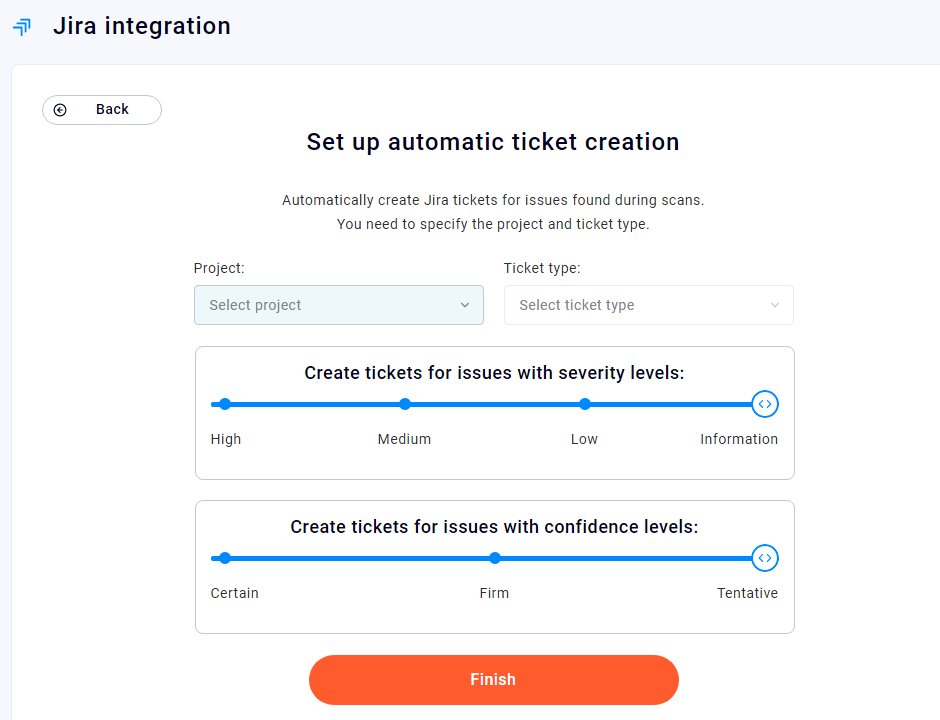The image features a user interface from the Jira application, predominantly shaded in light and standard blues. Along the top is a blue rectangular header with a very thin blue line underneath it. In the upper left-hand corner, within a light blue section of the header, there are three blue arrows pointing towards the top and right, adjacent to the text "Jira operation" in black, followed by white space.

Beneath this header, the main section of the interface focuses on setting up automatic ticket creation for issues found during scans. Centrally positioned, it states: "Set up automatic ticket creation. Automatically create Jira tickets for issues found during scans. You need to specify the project and ticket type."

Below this instruction, there are selections for both "Project" and "Ticket type." Each is displayed within a blue rectangle outlined in gray. The "Project" section contains the label "Select project" accompanied by a downward-pointing arrow on the right side. The "Ticket type" section similarly displays "Select ticket type" with an adjacent downward-pointing arrow.

Further down, there are configurable settings for ticket creation based on issue severity levels and confidence levels. 

The severity level configuration features:
- A gray outlined rectangle with the text "Create tickets for issues with severity levels."
- Below this, a horizontal blue line with three filled blue dots labeled "High," "Medium," and "Low."
- At the end of this line is a larger blue outlined dot with arrows pointing left and right, labeled "Information."

For confidence levels:
- Another gray outlined rectangle reads "Create tickets for issues with confidence levels."
- Beneath this is a horizontal blue line with two filled blue circles labeled "Certain" and "Firm."
- At the end of this line is a larger blue outlined circle with arrows pointing left and right, labeled "Tentative."

At the bottom of the interface, an orange button with rounded sides, bulging slightly on the left and right, is labeled "Finish."

This detailed interface allows users to specify project, ticket type, issue severity, and confidence level for automatic ticket creation in Jira.